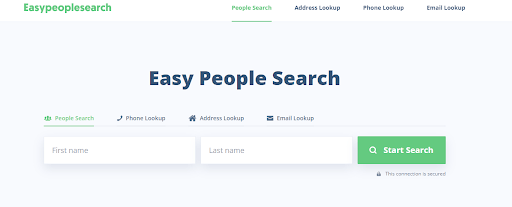The image shows the homepage of a website named "EasyPeopleSearch" displayed prominently in the upper left corner of the screen. The website name is styled in green, with no spaces between the words, and each word starting with an uppercase letter, making it "EasyPeopleSearch." 

Adjacent to the site name, a series of headings stretches from the center to the right of the screen. These headings include "People Search," "Address Lookup," "Phone Lookup," and "Email Lookup." The "People Search" option is currently highlighted in green to indicate it is selected, with a green highlighter underneath it.

The selection of "People Search" brings up a dedicated search interface in the middle of the screen, with the title "Easy People Search" displayed above it. This search section features two input fields for users to enter a person's first and last names. Below these fields, a green button labeled "Start Search" allows the user to commence the search process.

While "People Search" is highlighted and active, the other search options ("Address Lookup," "Phone Lookup," and "Email Lookup") are visible but grayed out, indicating they are not currently selected.